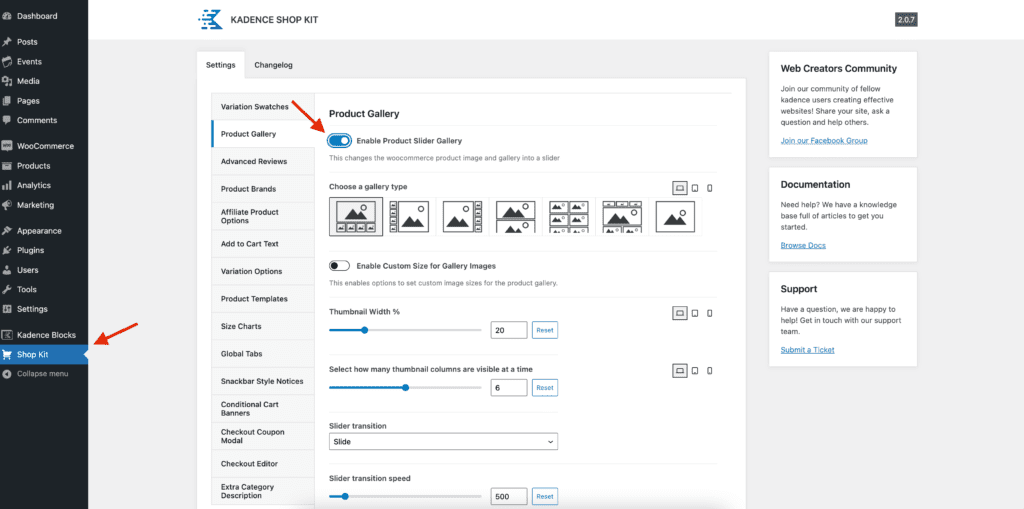In this image, we see a screenshot of a web interface set against a white and gray background. The upper left corner features the company name "Cadence" next to the "Shop Kit" logo, which has a stylized "K" to its left. Running vertically along the left side of the image is a black navigation bar with menu items listed in gray text. The menu items include (from top to bottom): Dashboard, Posts, Events, Media, Pages, Comments, WooCommerce, Products, Analytics, Marketing, Appearance, Plugins, Users, Tools, Settings, Cadence Blocks, and a highlighted "Shop Kit" at the bottom, accented with a blue background and a shopping cart icon. An attention-grabbing red arrow points directly to the "Shop Kit" option.

On the upper right corner, within a white rectangular box, there is a promotional message from the "Web Creators Community." The message reads: "Join our community of fellow Cadence users creating effective websites. Share your site, ask a question, and help others." Below this message is a blue hyperlink inviting users to "Join our Facebook group."